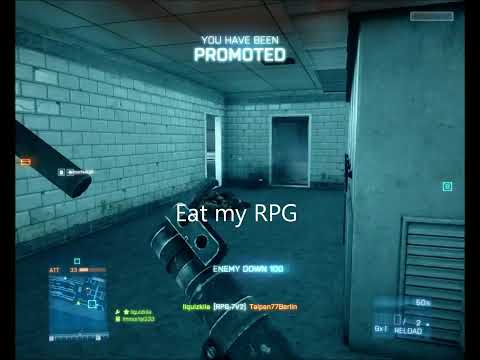This image is from a first-person shooter video game, featuring a dimly lit corridor with cement and white brick walls, and a ceiling resembling office tiles. At the right corner, there's a noticeable AC vent near the floor. The player’s point of view shows a large cannon-like gun in the process of reloading, and only the weapon is visible to represent the player. The scene is cast in dark green to bluish hues, indicating poor lighting typical of a warehouse or prison setting. 

Two doorways are open at the far end of the corridor, one on a wall directly ahead and another on the adjacent side wall to the left. On the bottom left of the screen, a mini-map guides the player's navigation. Prominent text overlays the scene: "You Have Been Promoted" at the top and "Eat My RPG" in the middle, signaling achievements in the game. Additionally, the phrase "Enemy Down 100" in a white font indicates a score for eliminating an enemy who is now visible lying on the ground in front of the gun. The corridor's atmosphere and the scattered in-game text contribute to a tense and immersive gameplay experience.